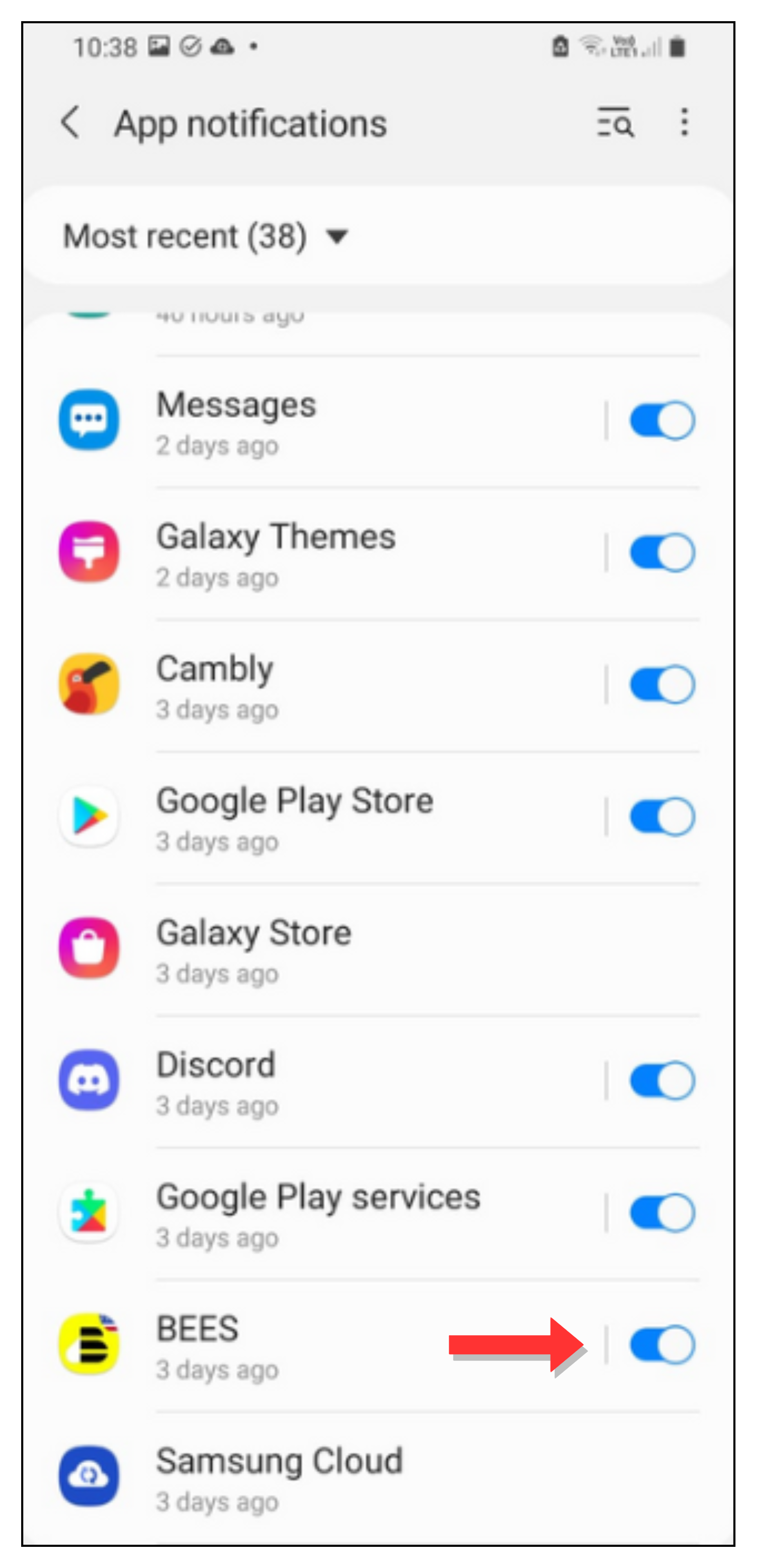Screenshot of App Notification Settings on a Cell Phone

The image captures the app notification settings screen on a mobile device. At the top-left corner, the time is displayed as 10:38, accompanied by various status icons such as signal strength and Wi-Fi. On the top-right, there are icons for battery status, service strength, and additional indicators.

The main title of the screen reads "App notifications," with a back button to its left and a search icon to its right. Directly below the title, there is a drop-down menu labeled "Most recent (38)."

Listed below are several apps: Messages, Galaxy Themes, Cambly, Google Play Store, Galaxy Store, Discord, Google Play Services, Bees, and Samsung Cloud. Each app, except for Galaxy Store and Samsung Cloud, has a switch next to it to toggle notifications on or off. The switches for all apps are in the 'on' position, except those without switches.

A prominent red arrow points horizontally towards the notification toggle switch for the 'Bees' application, drawing attention to this specific setting. Beneath each app name, a timestamp indicates the last interaction or notification received, such as "3 days ago" or "2 days ago."

This screenshot illustrates how users can manage notification settings for individual apps, with a particular focus on adjusting notifications for the Bees application.